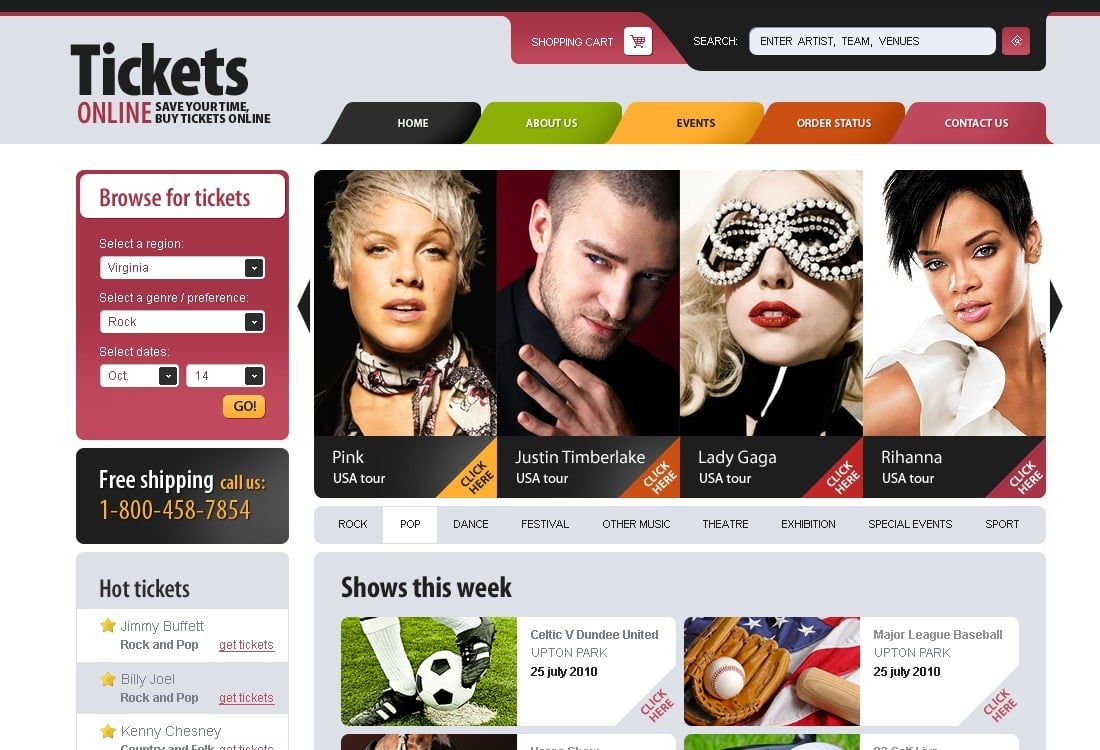This is a detailed screenshot from the TicketsOnline website. 

The interface features a gray header with a distinct mix of elements, including a small maroon tab labeled "Shopping Cart" and a search section with a black background. Adjacent to the search bar is a prominent red button. The header itself displays multicolored navigational tabs: "Home" in black, "About Us" in green, "Events" in yellow, "Order Status" in orange, and "Contact Us" in pink. 

The main content area highlights a dynamic slider showcasing four images of famous artists on their USA tours. The first slide promotes Pink, followed by Justin Timberlake, Lady Gaga, and Rihanna. Each slide is accompanied by a multicolored "Click Here" banner located at the bottom right of the photographs, inviting users to learn more.

Beneath the image slider, there is a section titled "Shows This Week," featuring upcoming events. The first listed event is a soccer match between Celtic and Dundee United at Upton Park on July 25, 2010. The second event is a Major League Baseball game also scheduled for July 25, 2010, at Upton Park, illustrated with an image of an American flag, a baseball mitt, a bat, and a baseball.

On the left-hand side, three additional sections provide more options and information:

1. **Browse for Tickets**: This section includes a region selector, a genre preference option, and date selection, all accompanied by an orange-gold button for search functionality.
   
2. **Free Shipping**: Featuring a telephone number for customer service.

3. **Hot Tickets**: Highlighting the most sought-after tickets available on the website.

This comprehensive layout and design focus on providing users with an intuitive and engaging experience while browsing tickets for concerts, theater exhibitions, sports, and special events.